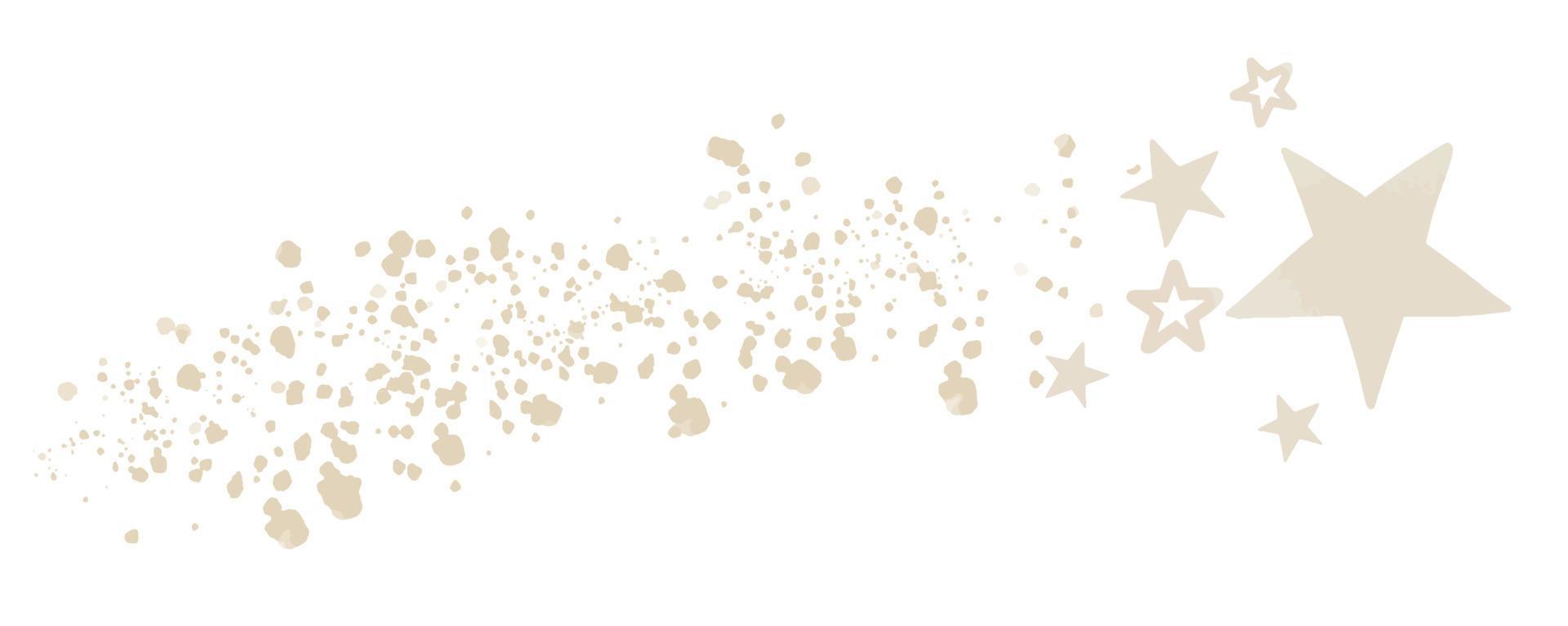In this hand-drawn or hand-painted illustration, a large ivory or cream-colored star dominates the right side against a white background. Surrounding this prominent star, to its left, are five smaller stars: two are outlined and three are completely filled in with the same opaque cream color. These stars form a semi-circle around the large star. Further to the left, a trail of irregularly shaped dots or star dust, in a slightly darker shade, stretches across the image, suggesting movement from left to right. The arrangement and detailing evoke the sense of falling stars or an asteroid belt trailing across the clear expanse.